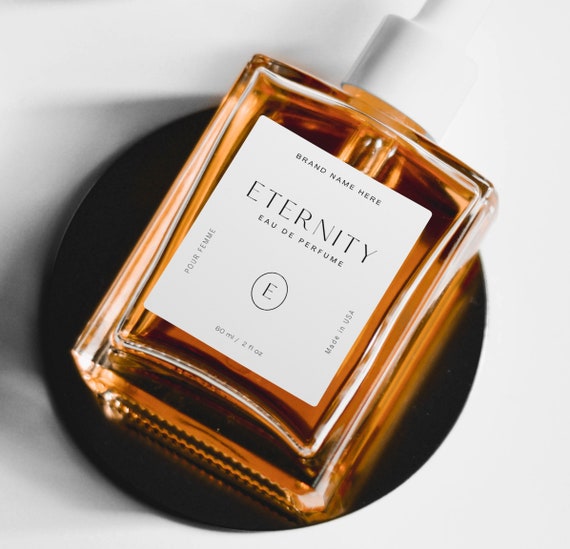This advertising image showcases a sample bottle of perfume called "Eternity." The bottle is positioned diagonally on a black disc that is set against a white surface. The bottle itself is made of clear glass, allowing the viewer to see the dark, amber-colored perfume inside. The design of the bottle is quite plain and square-shaped, with a simple off-white label at the center. The label features the text "brand name here" at the top, followed by "Eternity Eau de Parfum" in capital letters, and further down, it indicates “60 milliliters / 2 fl. oz.” In addition, there is a circled capital letter "E" on the label, hinting at a placeholder for branding. The bottle is topped with a white plastic screw-on lid, resembling the top of an ointment bottle, which emphasizes its status as a sample product rather than a final, retail version. The overall lighting illuminates the perfume, highlighting its rich color, while the plain presentation underscores its role as a mock-up design.